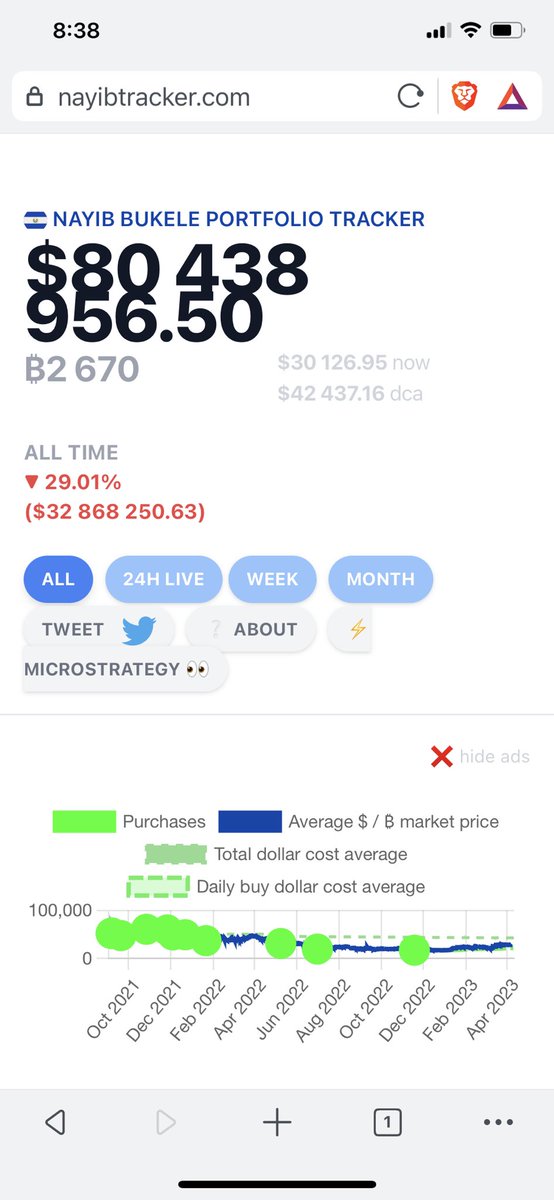**Detailed Caption:**

The image appears to be a screenshot taken from a smartphone, showcasing a website named naibtracker.com, dedicated to tracking the portfolio of Nayib Bukele. At the bottom of the screen, there is a navigation bar with a highlighted back arrow, indicating it can be pressed but not currently functional to move forward, likely because the user hasn’t navigated further yet. To the right of the back arrow are three more icons: a plus button, a box symbol, and three vertical dots for additional options.

Directly above this navigation bar, there are additional website controls: a refresh button, a lion icon, and a triangle symbol. The time displayed at the top of the screen is 8:38, with the battery life and Wi-Fi signal strength shown in the upper right corner.

The site interface indicates a focus on stock tracking. Below the search field and along the top section, "NAIB BUKELE PORTFOLIO TRACKER" is prominently displayed in blue. The portfolio’s current value is listed as 80438, with additional values of 95650.50, B2670, and a faded figure of 30,126.95. Another figure, 42,437.16 DCA, indicates all-time performance and is trending downwards in red by 29.01%, followed by additional numerical data in parentheses.

The interface includes a blue button offering views of "All," "24 hour," "Live," "Week," and "Month" data. There is also a tweet button related to "Lightning." The graphical display presents current stock prices marked with different purchase indicators in green, blue, and other colors. The timeline of the displayed data ranges from October 2021 to April 2023.